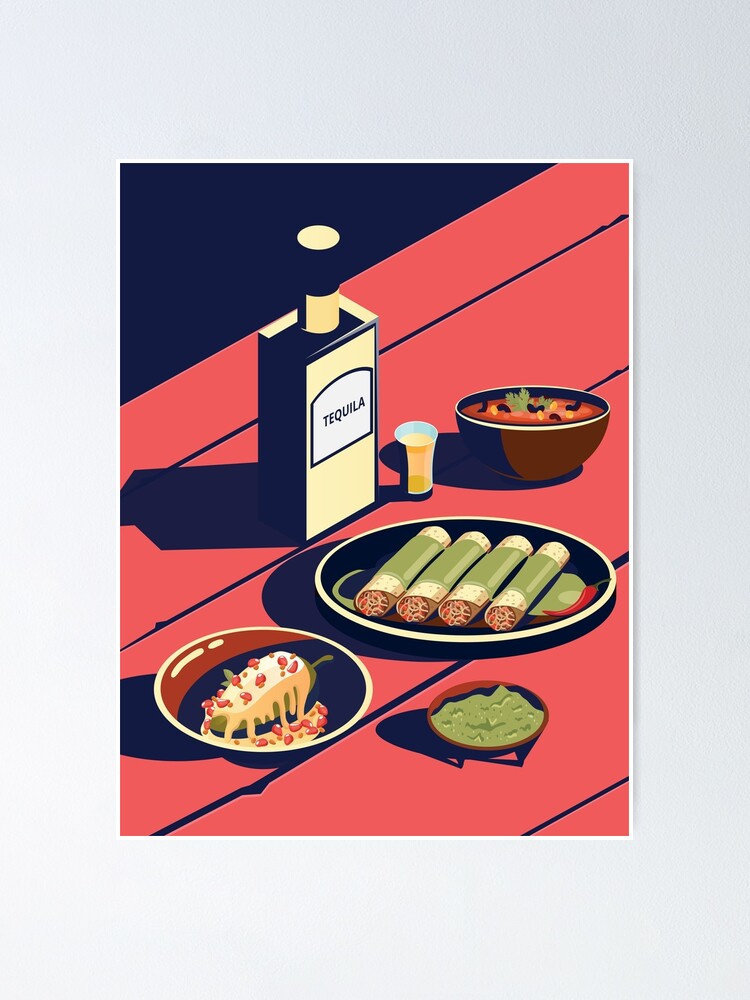This artwork depicts a vibrant spread of Mexican cuisine arranged on a diagonally-planked, red-painted wooden table. At the forefront, a bottle of tequila with a white label stands prominently, accompanied by a shot glass filled with bright yellow tequila. In the center of the table lies a plate of enchiladas, rolled into neat tubes and generously coated with green sauce. Nearby, a dish brimming with rich, red soup featuring green leaves and beans adds a splash of color. To the right, a guacamole dip sits invitingly with its creamy green texture, while a plate of cheese-covered poblano peppers, adorned with diced tomatoes, adds visual interest with its beige and red accents. The detailed artwork captures the essence of a festive outdoor meal, harmonizing the elements of traditional Mexican fare in a single appetizing tableau.